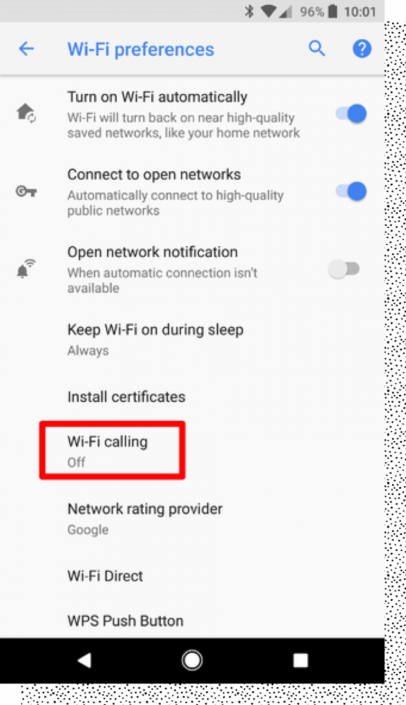The image displays a website open on an iPhone, captured at 10:01 AM with a battery life of 96%. The connectivity bar is halfway filled, indicating a moderate connection strength. At the top, in large blue letters, it reads "Wi-Fi preferences," accompanied by a blue arrow pointing left. Adjacent to this, a blue search icon and a circular help icon with a question mark are separated by a light gray line.

Below are several Wi-Fi settings:
- "Turn on Wi-Fi automatically" is enabled, indicated by a blue round slider.
- "Connect to open networks" is also turned on, with an illuminated blue slider.
- "Open network notification" is turned off.
- "Keep Wi-Fi on during sleep" is set to "Always."
- A section for installing certificates.
- "Wi-Fi calling" is off, highlighted by a red button outline.
- "Network rating provider," listed as Google.
- "Wi-Fi Direct" and "WPS push button" options, followed by a thick black bar at the bottom.